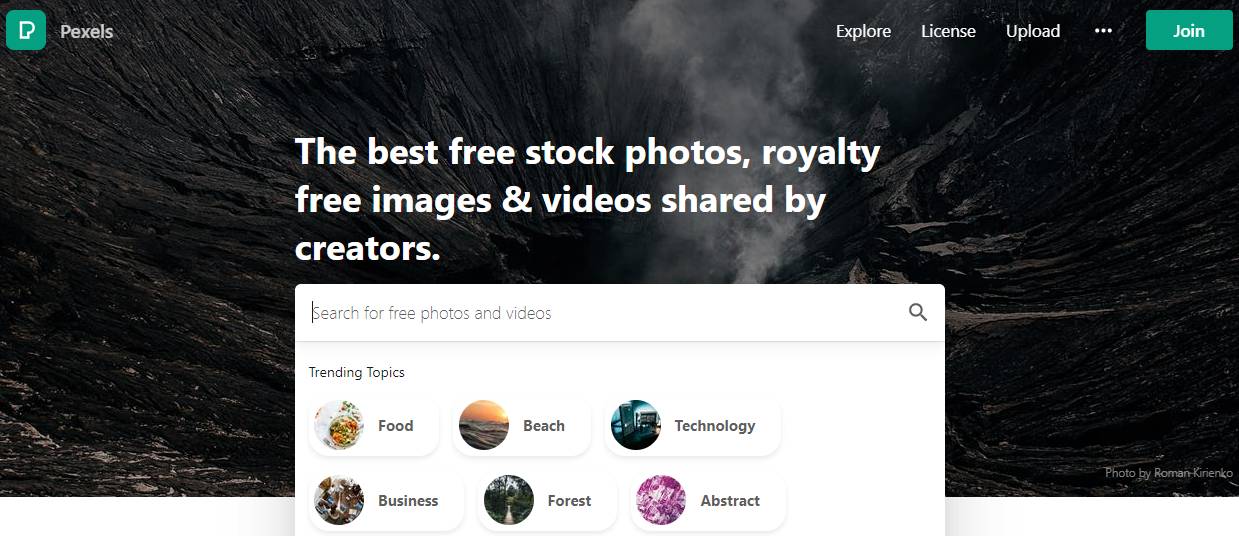A high-angle photograph showcases the dramatic landscape of a volcanic area, characterized by a deep, smoke-emitting crater. The terrain is rugged and predominantly black, reinforcing the raw, untamed nature of the scene. In the top left corner of the image, there is a teal square with a white outline of the letter "P," followed by the word "Pexels" to its right. On the upper right side of the image, the words "Explore," "License," "Upload," and an ellipsis are displayed, accompanied by a teal button labeled "Join." Below this button, white text reads, "The best free stock photos, royalty-free images, and videos shared by creators." Additionally, a search box with the placeholder text "Search for free photos and videos" and a magnifying glass icon is visible. Beneath the search box, popular trending topics such as "Food," "Beach," "Technology," "Business," "Forest," and "Abstract" are listed.